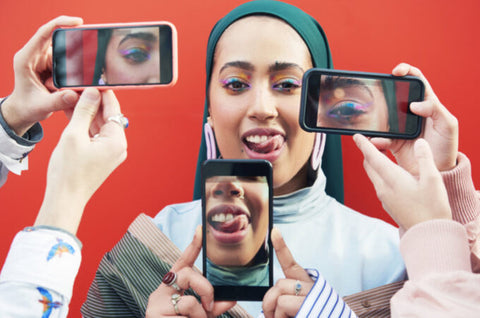This captivating image features a young woman, possibly of Somali descent, adorned in a vibrant green headscarf and a striped outfit. She wears bright blue and pink eye makeup, and her mouth is playfully open with her tongue out to the side. Her face is embellished with earrings and rings, adding to her vivid appearance. Holding her own phone, she captures a selfie that focuses on her mouth. Beside her, two other individuals, likely also female, are engrossed in photographing her eyes—one focusing on her left eye and the other on her right. The scene is lively, capturing a moment of fun and camaraderie as they meticulously document the intricate details of her colorful makeup.